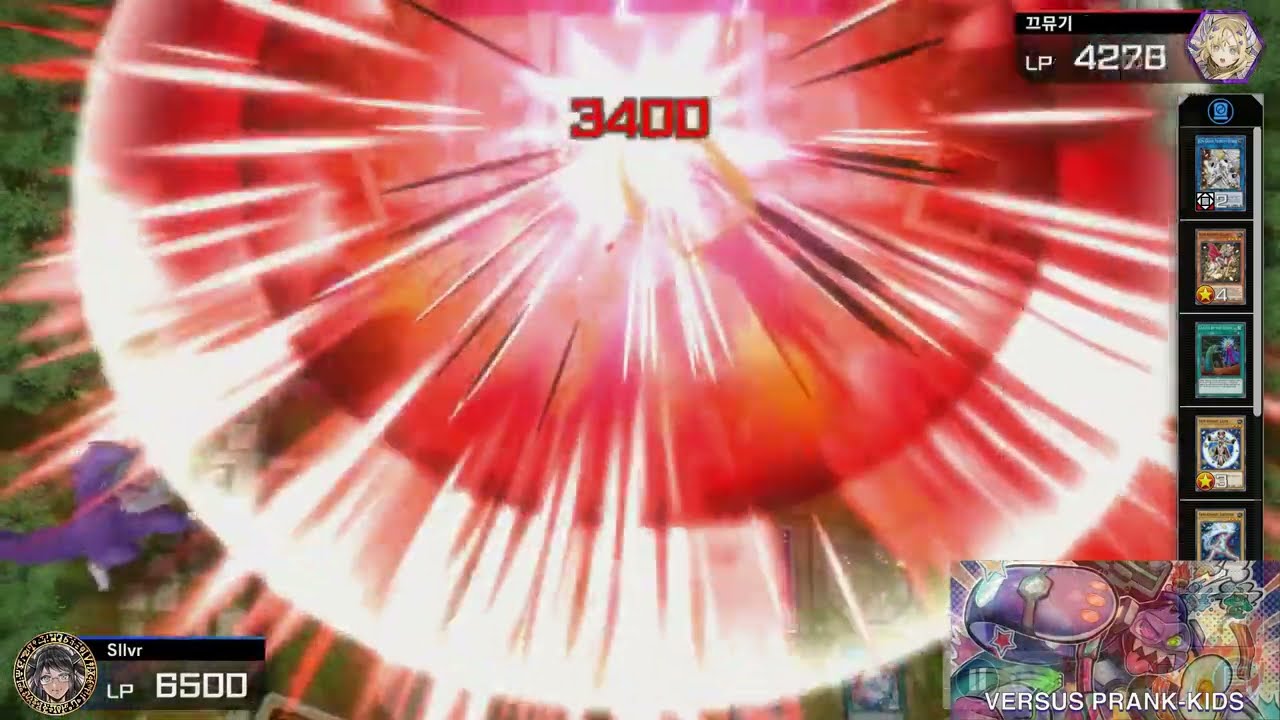This image is a detailed screenshot from a video game, likely a digital card game resembling Yu-Gi-Oh. At the center of the image, a dramatic explosion radiates red and white beams, prominently displaying the number "3400" in red. In the upper right corner, there's text labeled "LP4278" alongside a character embedded within a hexagram. The bottom left corner showcases an avatar or player icon, labeled "SLLVR," with the text "LP6500" in white underneath it. The game's graphical interface indicates a match, as denoted by a pop-up box on the bottom right corner, which reads "versus prank-kids," accompanied by graffiti-style imagery. Additionally, the far right side of the screen features card-like elements with numbers and different colored images, reinforcing the card game theme. Overall, the setting is cartoony and vibrant, featuring a wide palette of colors, including red, white, brown, yellow, blue, purple, pink, and green.